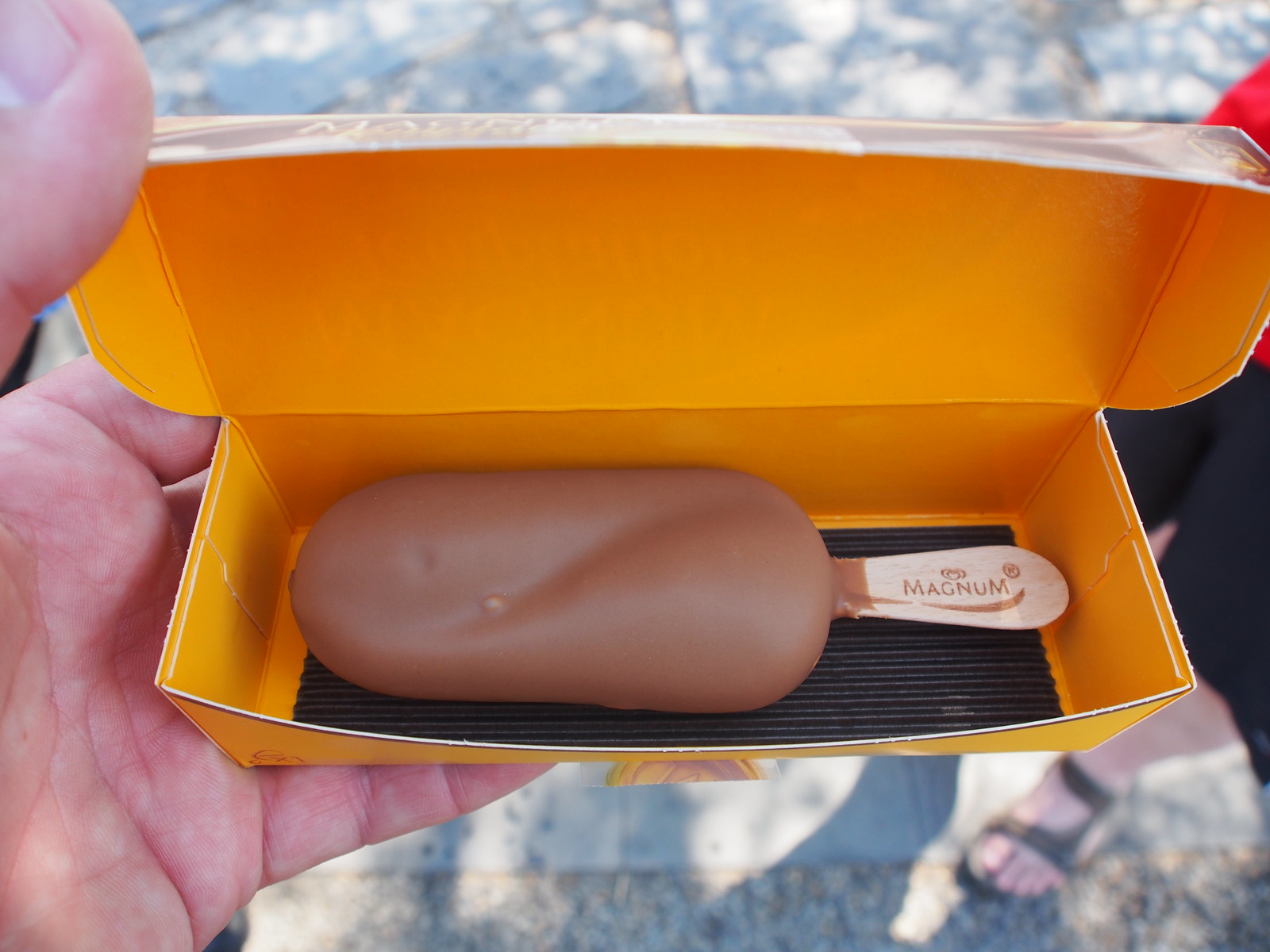A close-up image captures a man's left hand holding a partially open container that resembles a corndog box with a black base and an all-orange interior. Inside the box sits a chocolate-covered ice cream bar, branded "MAGNUM" with the name engraved in capital letters on its wooden stick. The ice cream bar has a slight dent in the middle of its glossy chocolate shell. In the background, on a sunlit sidewalk, stands another person wearing sandals, black shorts, and a red shirt. The evening light casts long shadows, adding to the casual, outdoor atmosphere.